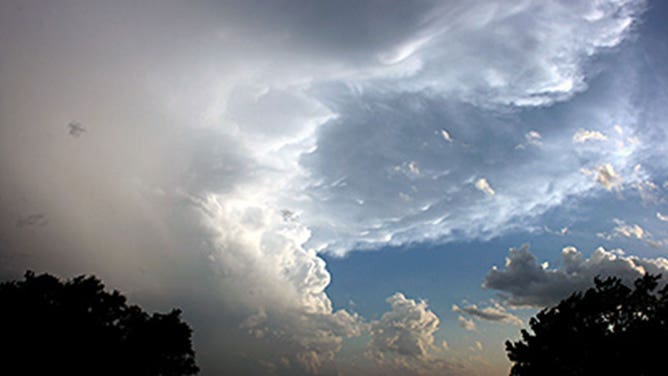The image captures a tumultuous sky, suggesting the onset of a storm or possible tornado. Dominating the scene are large, varying shades of clouds, from bright, shining whites to ominous dark grays and blacks, with hints of grayish-yellow strewn through. These clouds exhibit a jagged, billowy, and fluffy appearance, with the darker ones swirling and forming a point towards the top, giving the impression of a funnel or tornado-like form. The sky opens up to a vivid blue in the bottom right, where the sun casts its light, creating contrasting illuminations on the cloud surfaces. Nestled in the bottom left and right corners of the image are the tops of two lush trees, their large leaves in full bloom, grounding the chaotic sky scene.